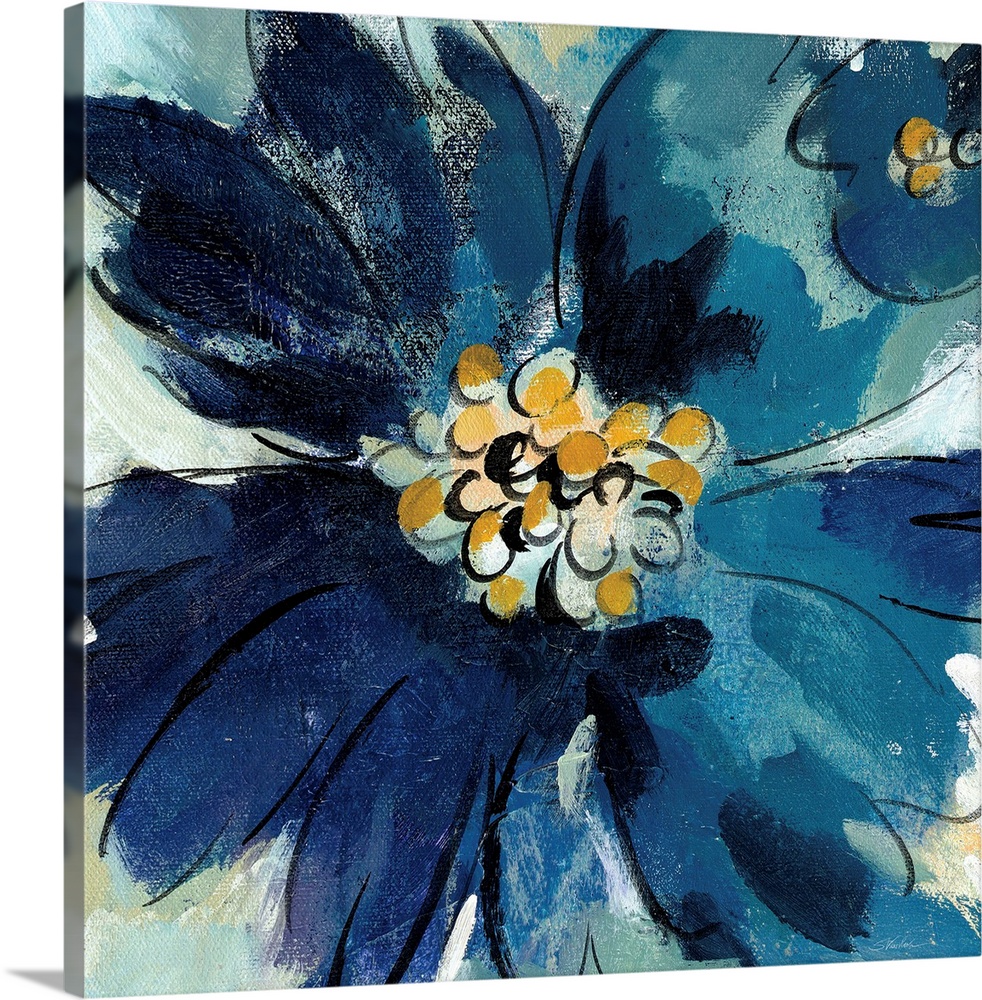This image is a color photograph showcasing a canvas painting of a flower, positioned against a white background that includes a subtle shadow, suggesting it is displayed on a flat surface. The canvas itself is fully visible, including its side borders. The flower dominates the painting with intricately detailed petals outlined in black. The petals exhibit a gradient of blue hues, ranging from dark blue on the left to lighter blue on the right, some with hints of green and black tinges. The central part of the flower is vibrant yellow with several yellow and white circles, some blurred and all outlined in black. In the upper right corner, a smaller, partially visible flower features two yellow circles at its center. The entire composition conveys an abstract aesthetic. Notably, the painting is unsigned and undated.